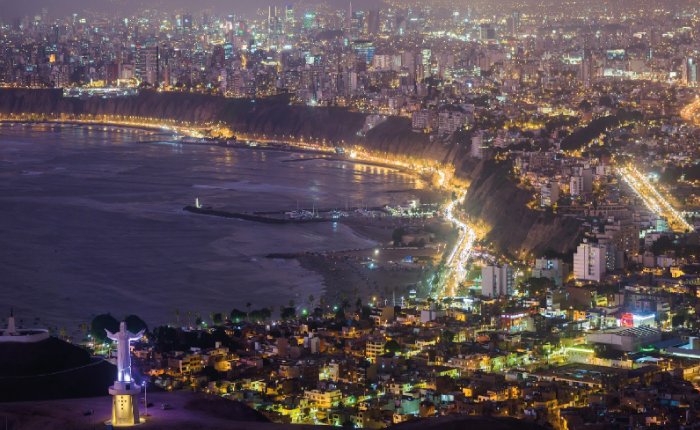The image captures an aerial nighttime view of a vibrant city, presumably Rio de Janeiro. The city is adorned with countless lights emanating from buildings of various sizes and busy streets. On the left side, the coastline is illuminated, suggesting a road that traces the water’s edge, accompanied by the headlights of numerous cars. Adding to the spectacle is a prominent white statue with outstretched arms in the bottom left, reminiscent of Christ the Redeemer and hinting at the city's identity. The shoreline features a dramatic drop-off, perhaps a cliff, and a jetty extending into the bay. The right side showcases possibly several large buildings that could be hotels, their lights contributing to the glittering cityscape below.